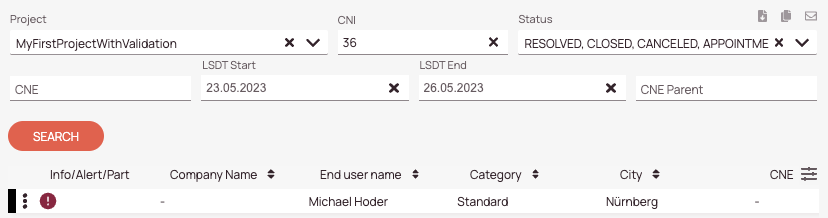A detailed screenshot of an app interface, likely from the backend of a form field validation system, is depicted. The image showcases various fields and options, including a project titled "My First Project with Validation." Users can resolve, close, or cancel the appointment. Key fields include "Status," "CM," and "CME Field," along with a timestamp. There is a distinct orange button labeled "Search," and a highlighted white section that displays the name "Michael Holder." Additionally, the app mentions "Standard" and "Numburg," potentially denoting categories or additional criteria. The interface appears to be designed for managing and validating project details efficiently.